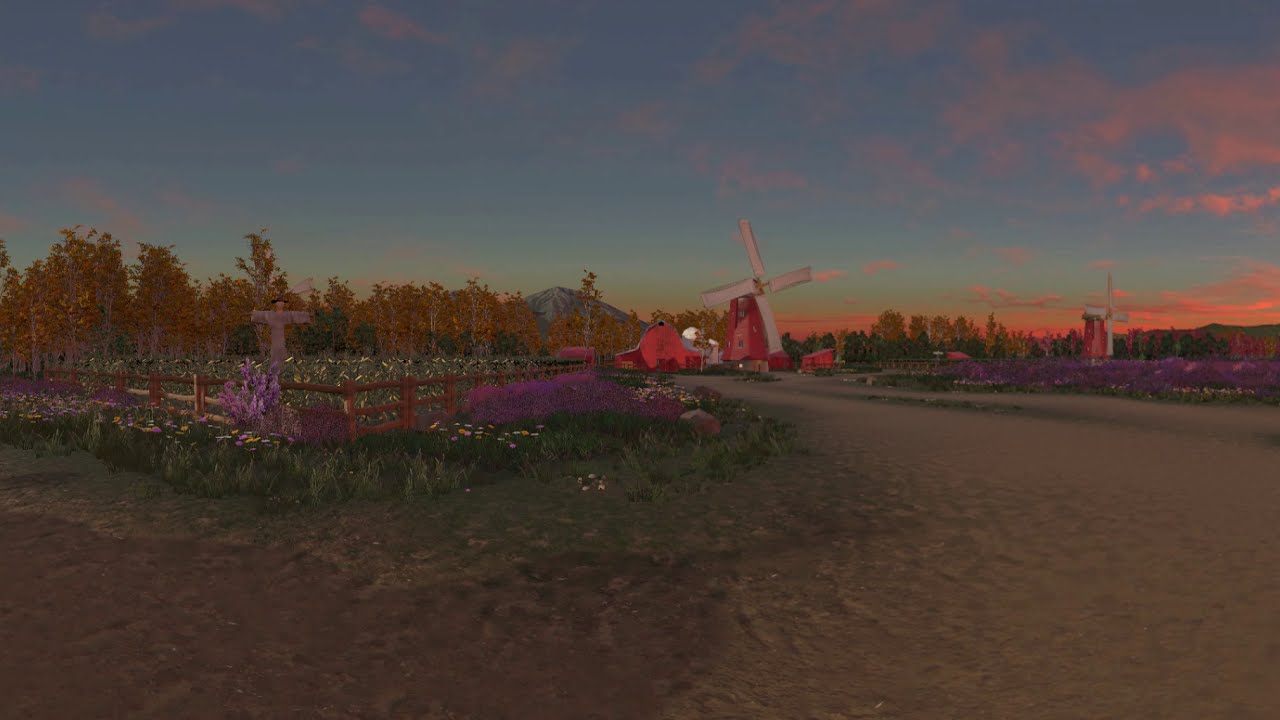This captivating painting depicts a serene sunset scene on a farm, characterized by warm orange and deep blue skies, tinged with sunset hues. The setting is a pastoral field with patches of grass, vibrant purple flowers, and soil. Dominating the scene are two old-style red windmills with white fabric fan blades, one positioned centrally and the other in the background to the right. They are complemented by a large red and white barn, exuding rustic charm. To the left, a fenced-off garden area with a scarecrow provides additional quaintness. Behind the structures, a dense line of green trees stretches across the horizon, while the peak of a distant mountain or volcano looms majestically in the background. The overall ambiance, enhanced by the play of dusk light and the tranquil rural elements, suggests the scene could either be a detailed painting or a realistic depiction within a video game.